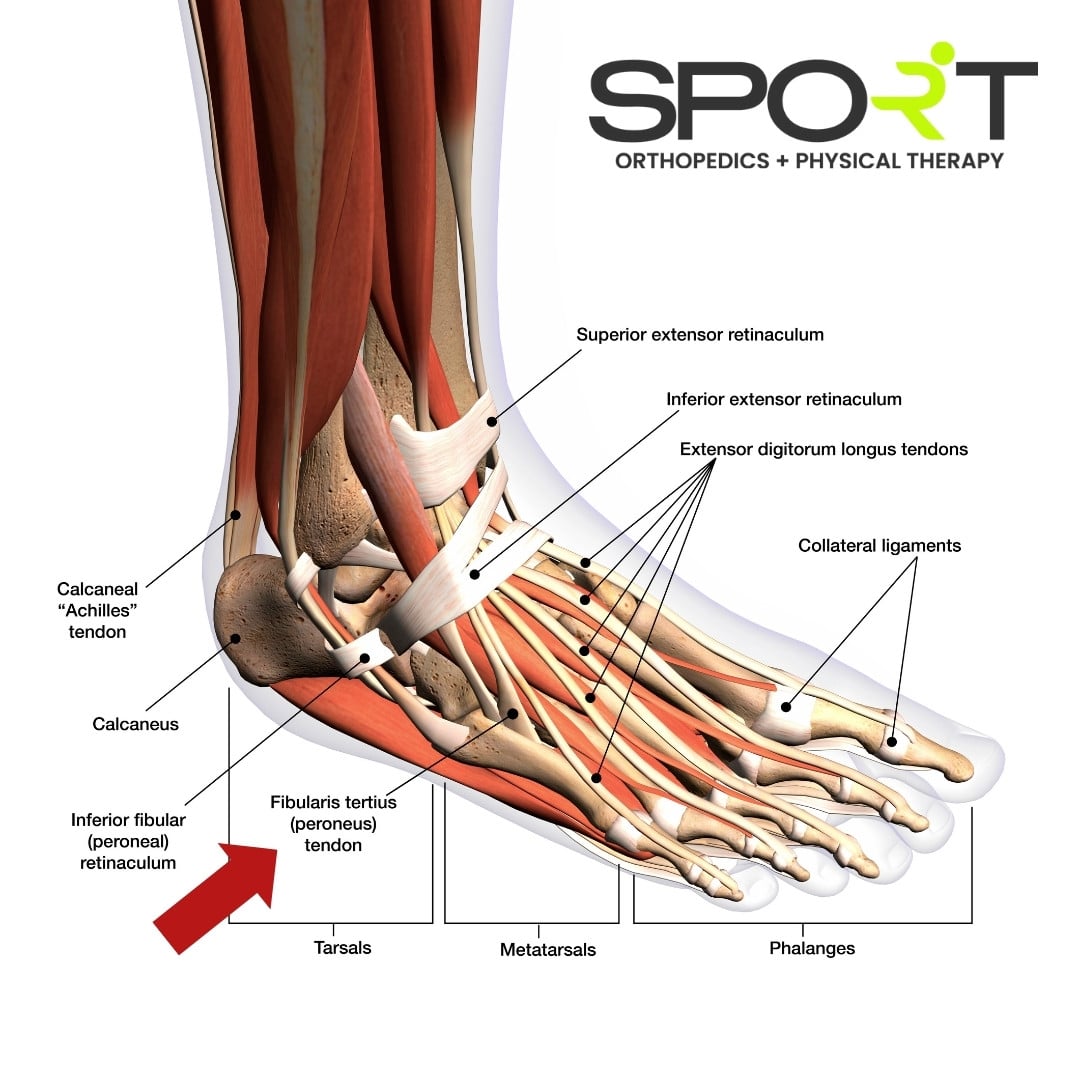The image with a plain white background illustrates a detailed anatomical diagram of a right foot and lower ankle, specifically highlighting the skeletal and muscular structures. At the top right corner, the title "Sport Orthopedics + Physical Therapy" is displayed, where the "R" in sport is depicted in green to resemble a skater in motion. The diagram includes labels and black lines pointing to various parts of the foot, such as the superior and inferior extensor retinacula, extensor digitorum longus tendons, collateral ligaments, and key bones, including the phalanges, metatarsals, and tarsals. The Achilles (calcaneal) tendon and fibularis tertius (peroneus) tendon are also identified. Additionally, a red arrow indicates specific structures at the bottom part, further detailing the tarsals, metatarsals, and phalanges.